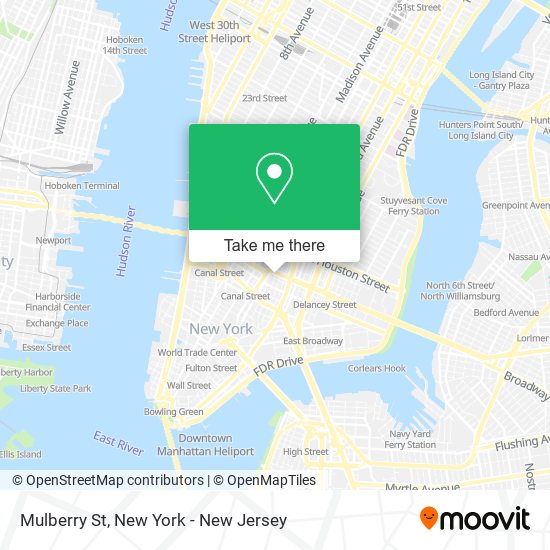This rectangular image, oriented vertically, features a detailed map of Manhattan with portions of Brooklyn and New Jersey visible. The map clearly highlights bodies of water, with the Hudson River and the East River represented in blue. Major thoroughfares are depicted in yellow, while smaller streets are shown as white lines.

Overlaying the map is a pop-up window that includes a blue button labeled "Take me there." Above this button, there is a smaller image featuring a street view of the highlighted location. This street view image includes buildings flanking both sides, crosswalks, a few cars, and an overcast sky.

At the bottom of the image, there are several labels: “OpenStreetMap contributors” and “OpenMapTiles,” along with the specific location “Mulberry Street, New York-New Jersey.” In the bottom right corner, the brand "Moovit" is displayed.